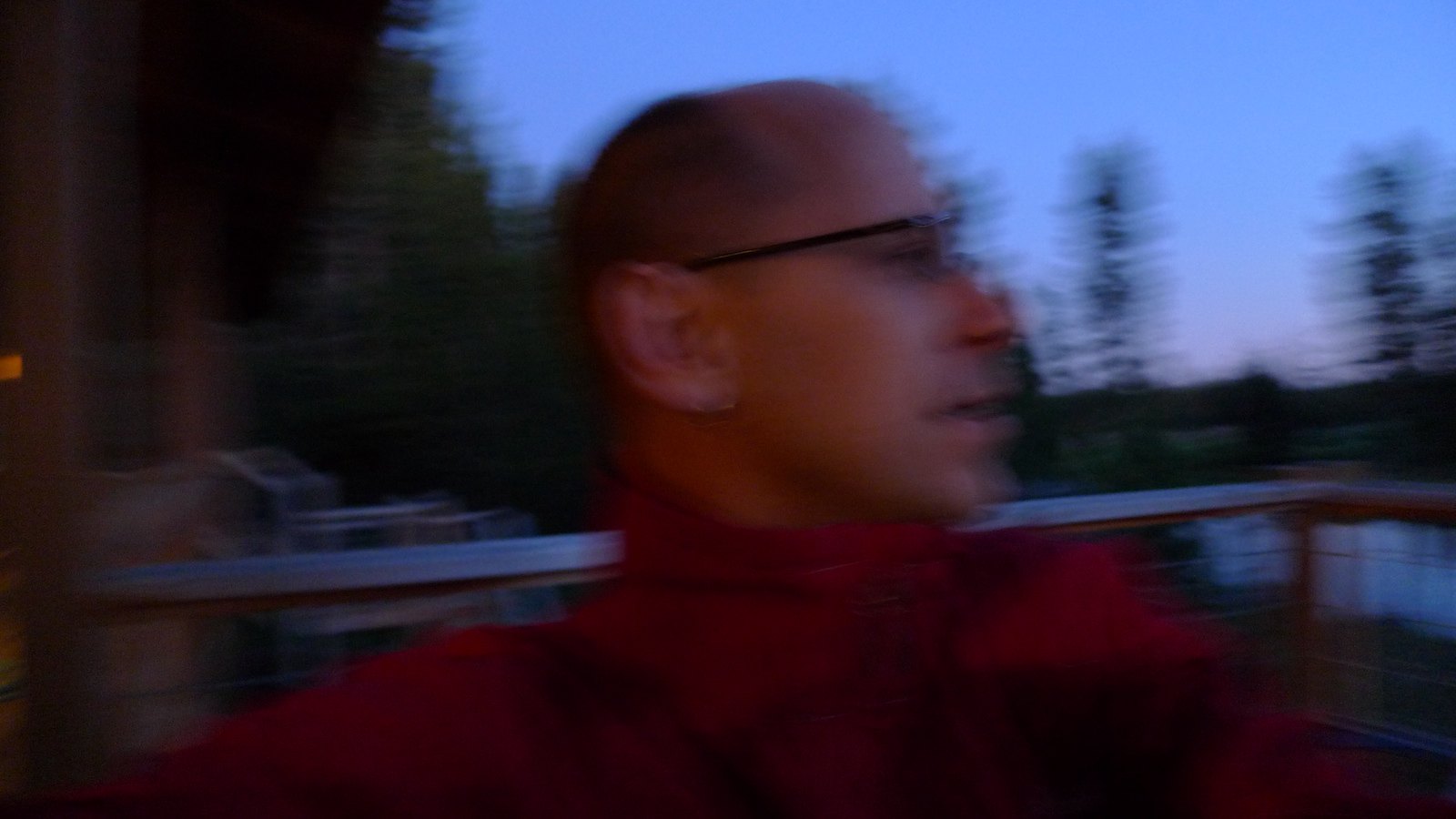The image is a slightly blurry color photograph of a man with short, balding hair and black glasses, viewed from the side, showing the right side of his face. He is wearing a red or burgundy long-sleeved sweater or jacket with a loosely gathered high neck. The setting appears to be an outdoor area, possibly a back porch in a forested region. Tall, narrow trees resembling pine trees and significant greenery feature prominently in the background. The sky is blue but dimming, indicating that it is around twilight, possibly 7:30 PM, with the sun having just set. The image's blurriness suggests it was taken while the camera was in motion. Additionally, there might be some water and a bridge visible, although this detail is unclear due to the image's lack of sharpness.